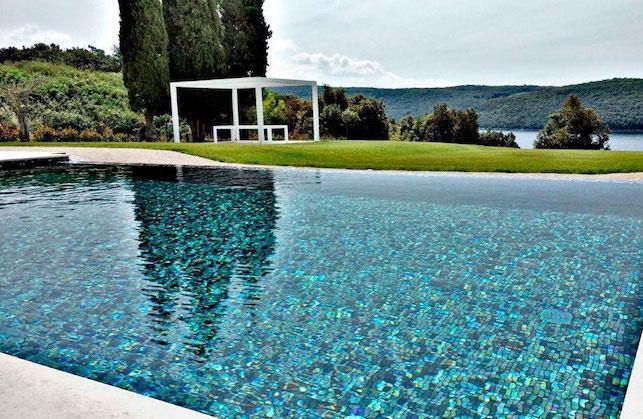A vibrant, terraced pool with a bottom lined in varying hues of blue and teal tiles dominates the foreground of the image, creating a stunningly vibrant blue appearance. The pool’s large tiled squares give it a textured look that appears almost like a mosaic. Sunlight bathes the scene, casting reflections of nearby trees onto the water, and accentuating the beauty of the clear blue sky dotted with large, fluffy clouds. 

In the background, a carefully manicured green space features a charming white gazebo, complemented by a white table and bench that add a quaint touch. Behind the gazebo, three tall conifer trees stand proudly, leading the eye to a large, tree-covered hill. Beyond this, the pool offers a breathtaking overlook of a vast lake, surrounded by an expansive landscape of hills and mountains cloaked in rich vegetation. The setting exudes serenity, suggesting an idyllic park or a luxurious backyard retreat.